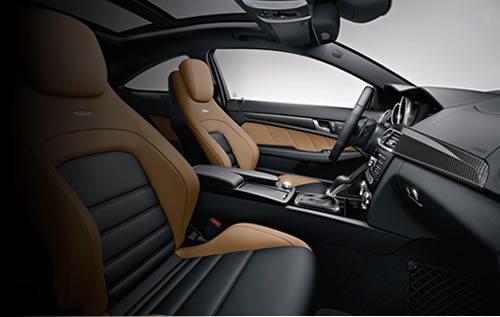The image captures the interior of a futuristic car, possibly an SUV or a large vehicle. The perspective is from the passenger seat facing the driver's seat and out the window, revealing a sleek and spacious design. The cabin features segmented black leather seats with brown trim and brown headrests. The expansive windshield, larger than in typical cars, suggests an open and airy feel and is accompanied by a moonroof or sunroof flanked by two clear panels. The details extend to the doors, which present trim that mirrors the supple leather of the seats, accented by wood-like or brown plastic paneling. Dominantly black, the interior is punctuated with silver detailing on the gear shift and center console, providing a modern touch. The photo captures both front seats, with the driver’s seat positioned farther away. The top of the vehicle showcases a pattern of white patches interspersed with black streaks. Additional details include visible glove box, floor mats, seat belt, armrest, and steering wheel, completing the minimalist yet luxurious look of the car's interior.